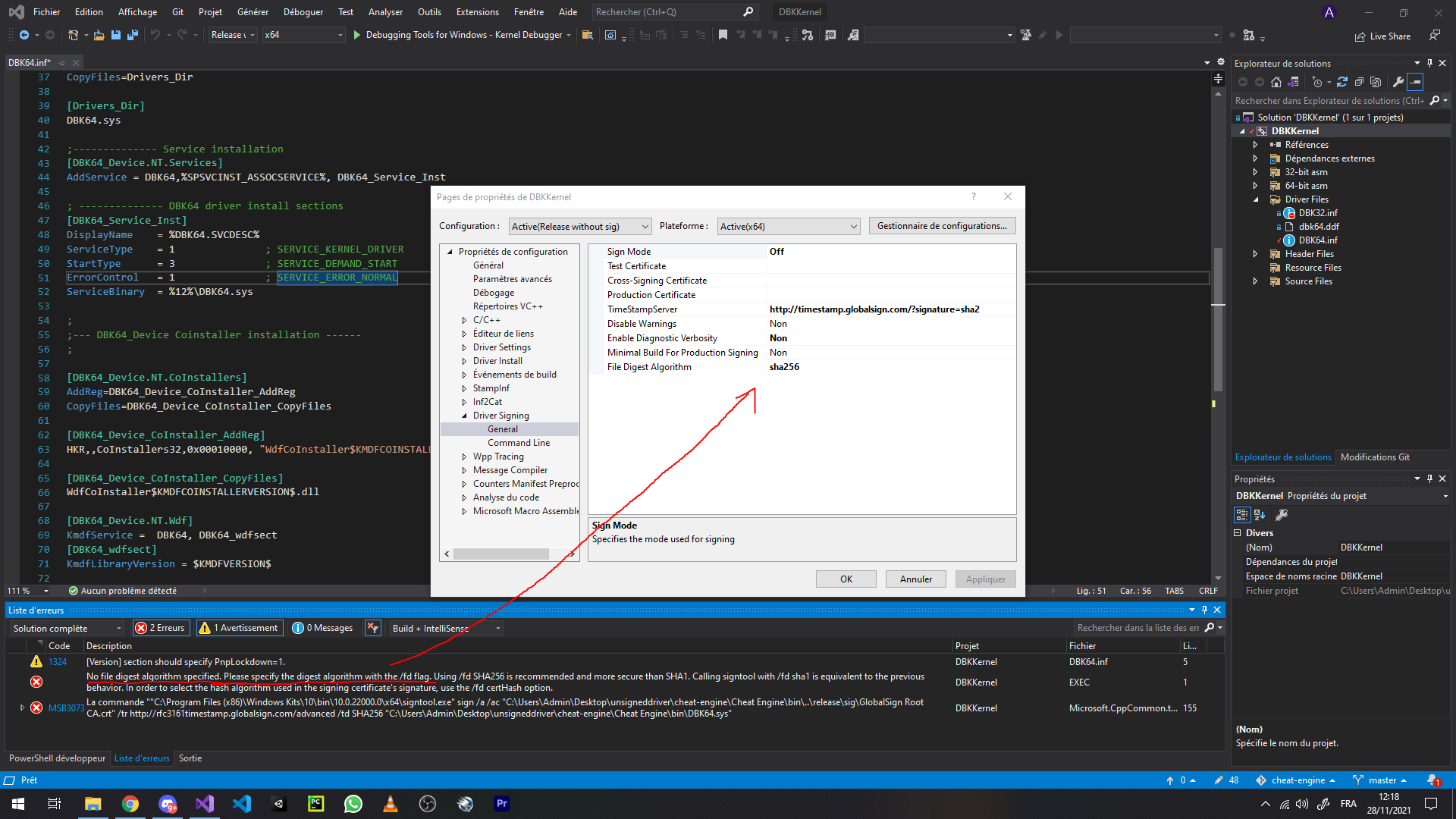A detailed screenshot of a computer screen, predominantly set in dark mode, features various open tabs and multiple coding panels displaying debug information. The central focus is a small white window, highlighted by a prominent red arrow. This window includes detailed configuration settings such as "Sign Mode: Off," "Test Certificate," "Cross-Signing Certificate," "Production Certificate," "Timestamp Server: http://timestamp.globalsign.com?signature?sha2," "Disable Warnings: Non," "Enable Diagnostic Verbosity: Non," "Minimal Build for Production Signing: Non," and "File Digest Algorithm: SHA-256." The red arrow specifically points to a black panel that contains a warning message: "No File Digest Algorithm Specified. Please specify the digest algorithm with the /fd flag." Above and around this central area, various colorful text snippets—greens and blues—are visible within the panes, indicating different sections of code. At the top of the screen, the viewer can see menu options labeled in what appears to be Dutch or German, including "fichier" (file), "addition," "affichage" (display), "JIT," and "project." Additionally, a blue toolbar is present at the bottom of the screen, along with the taskbar, completing the interface.